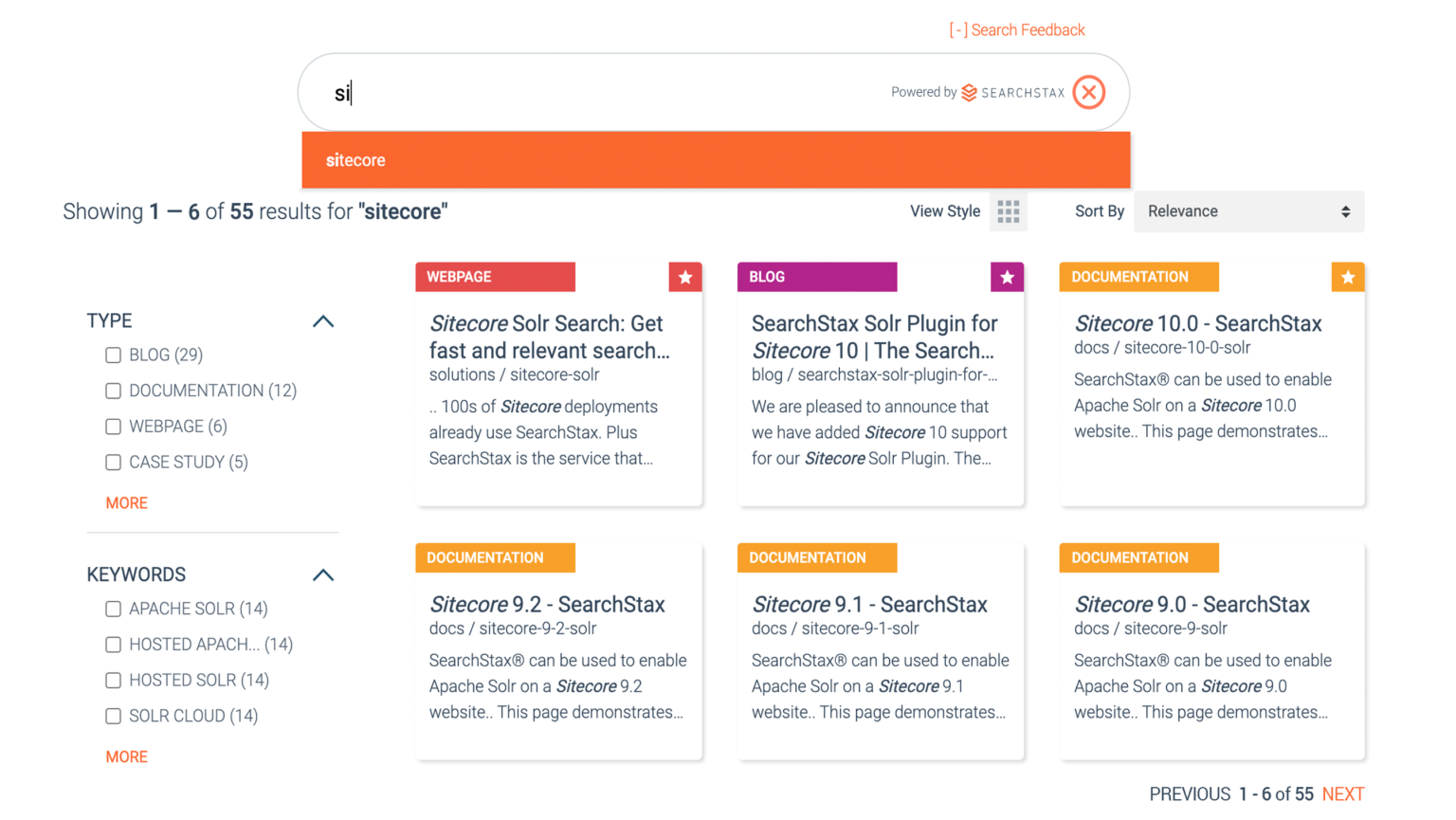The image displays a search interface branded as "Powered by Search Stacks," tailored for Sitecore queries. At the top, a search bar shows a user in the process of typing "SI," with Sitecore prominently appearing in an orange, rectangular highlight with white text. Beneath this, in black font, the interface indicates "Showing 1 through 6 of 55 results for Sitecore."

Users can toggle between grid and list views and sort results by relevance and other criteria. The search results are categorized, listing 29 blog posts, 12 pieces of documentation, 6 web pages, and 5 case studies related to Sitecore. An orange "More" button allows for additional exploration within these categories.

For keyword refinement, options include "Apache Solr," "Hosted Apache," "Hosted Solr," and "Solr Cloud," each expandable via a "More" button. The search results are visually presented in six small panels: one web page, one blog post, and four documentation entries.